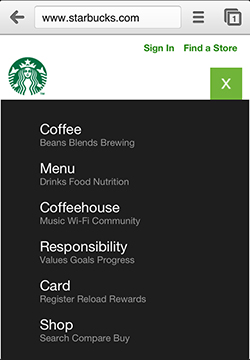The image showcases a detailed section of the Starbucks website interface, set against a light gray background. At the very top, a search bar is prominently featured with a small left-pointing arrow. Inside this search bar, the URL "www.starbucks.com" is displayed. To the right of the URL, there are three small horizontal lines, typically indicative of a menu, and a white square with the number "1" inside.

Directly below the search bar, the iconic Starbucks logo is centered, displaying the familiar mermaid with flowing, curvy lines that represent her hair, and her distinctive crown-like headpiece, all rendered in the classic dark green and white color scheme. To the right of the logo are green text options to "Sign In" or "Find a Store."

Beneath this, a green square houses a white "X". Following that, a long black rectangle lists several menu options in white text. The list begins with "Coffee" and subcategories like "Beans," "Blends," and "Brewing." The next main category is "Menu," followed by subcategories such as "Drinks," "Food," and "Nutrition." Further down, "Coffeehouse" is listed with subcategories including "Music," "Wi-Fi," and "Community." The list continues with "Responsibility" and subcategories such as "Values," "Goals," and "Progress." Further still, the "Card" category features options like "Register," "Reload," and "Rewards." The final main category is "Shop," with subcategories "Search," "Compare," and "Buy."